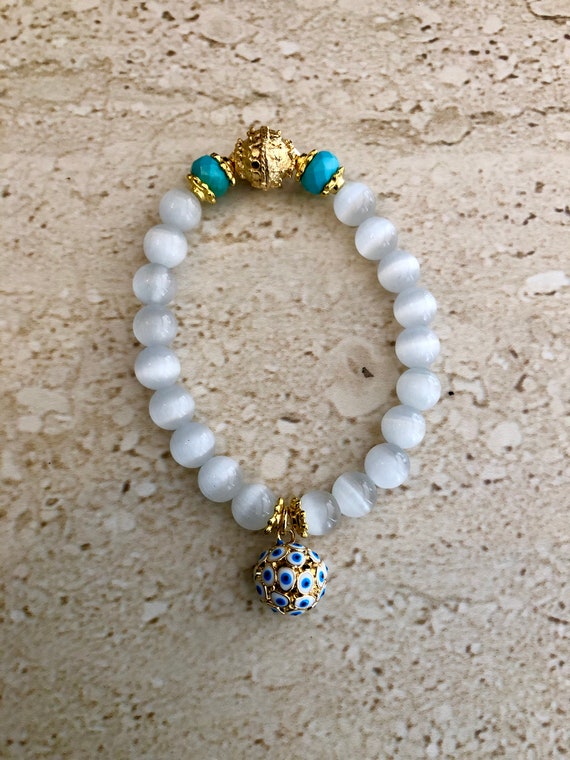The image captures a detailed close-up of a bracelet adorned with a variety of beads and intricate accents. The bracelet features predominantly white and clear beads that resemble pearls, interspersed with gold detailing. It rests on a white and gray marble countertop that has faint brownish patterns, adding a textured backdrop. At one end of the bracelet, a gold pendant dangles, adorned with small designs that resemble blue eyes with white and black detailing, giving it a striking focal point. At the opposite end, two turquoise beads are accented with gold framing, with a golden ball situated between them as a clasp. The overall effect is a harmonious blend of white, turquoise, and gold, with a slight blur in the background highlighting the bracelet's intricate features.